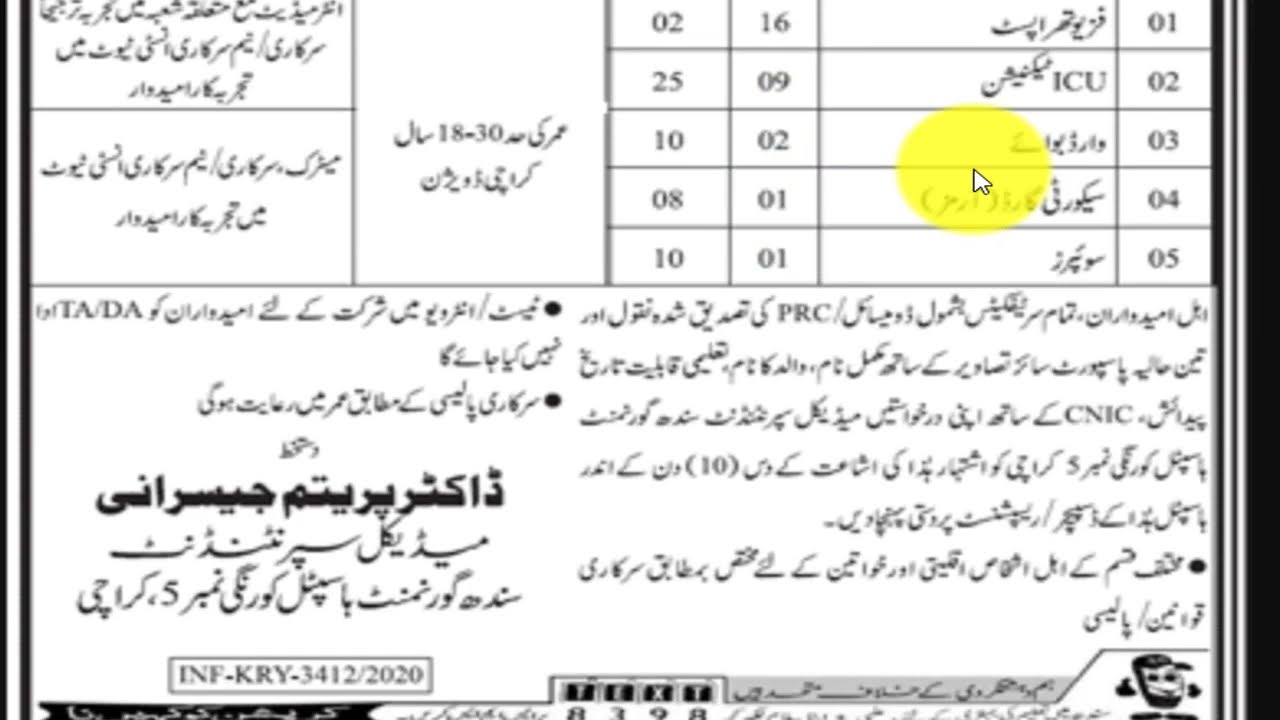The image appears to be a black-and-white photocopy or screenshot of a document, almost resembling a report or a legal document. The document is written in a non-Latin alphabet, possibly in Arabic, based on the cursive writing style and letter shapes. The document has a grid-like pattern at the top with visible numbers and is bordered by thick, dark black bands. Near the upper right-hand corner of the document, a mouse cursor points, and a large yellow circle highlights this section. Below the grid-like area, the bottom half of the document contains more text, where the font appears larger and distinct in places, possibly for emphasis. In the lower left-hand corner, there's a series of digits and letters: INF-KRY-3412/2020. The rest of the text and numbers are difficult to decipher.